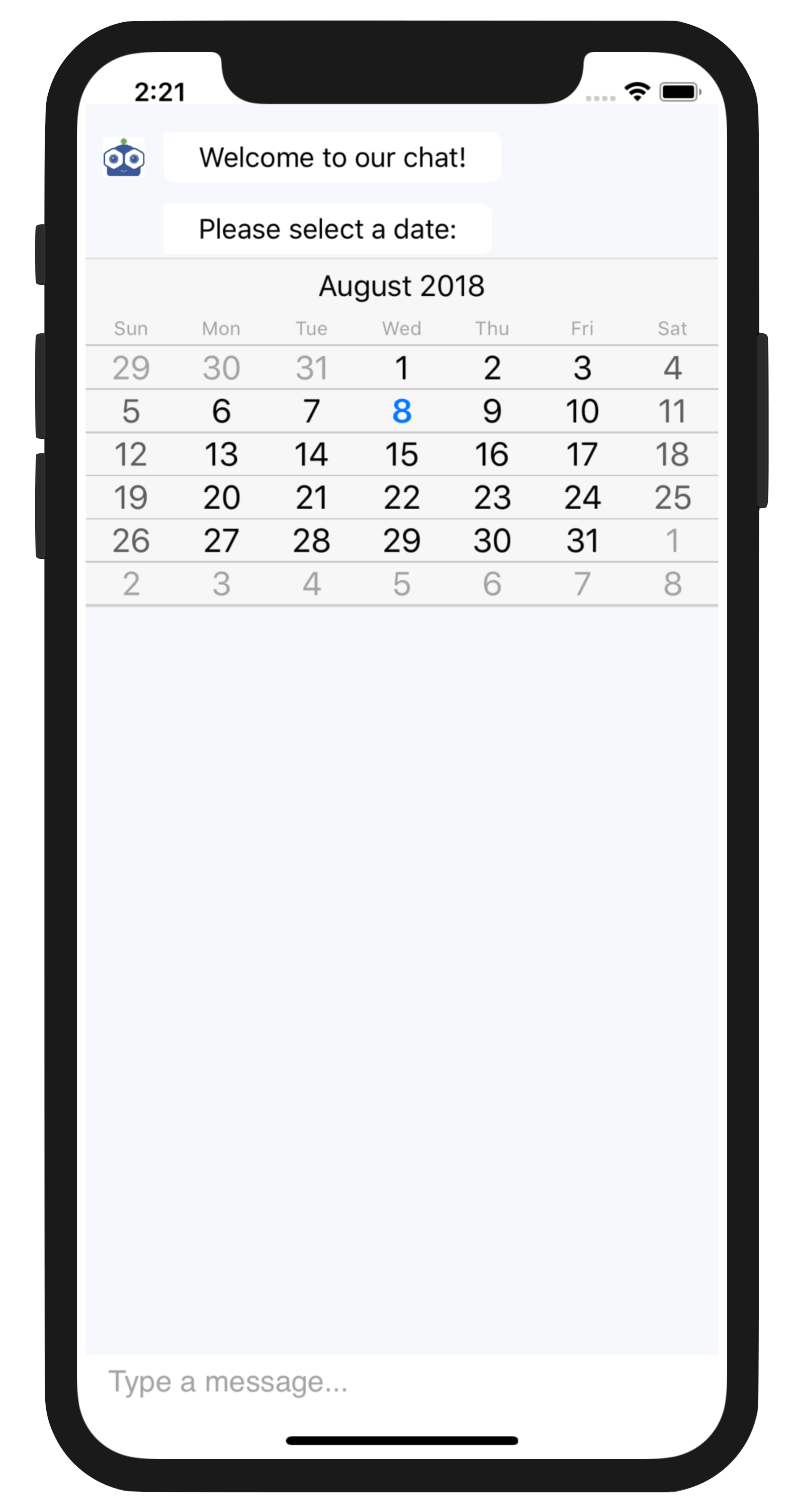The image depicts the screen interface of a cell phone. The phone has a black border surrounding a white display area. In the top left corner of the screen, the time is shown as "2:21." The top right corner displays three dots, indicating an options menu, a fully strong Wi-Fi signal icon, and an almost full battery icon.

Beneath these status indicators, there is a blue graphic depicting the top portion of a character's head and eyes. This graphic is associated with the message "Welcome to our chat."

Below this welcome message, the text prompts, "Please select the date," followed by the date "August 2018." Under the date prompt, there is a calendar layout for the month of August 2018, displaying the days and corresponding dates.

At the very bottom of the screen, the phrase "Type a message" is visible, and beneath it, there is a solid black line, possibly the input area for user text.